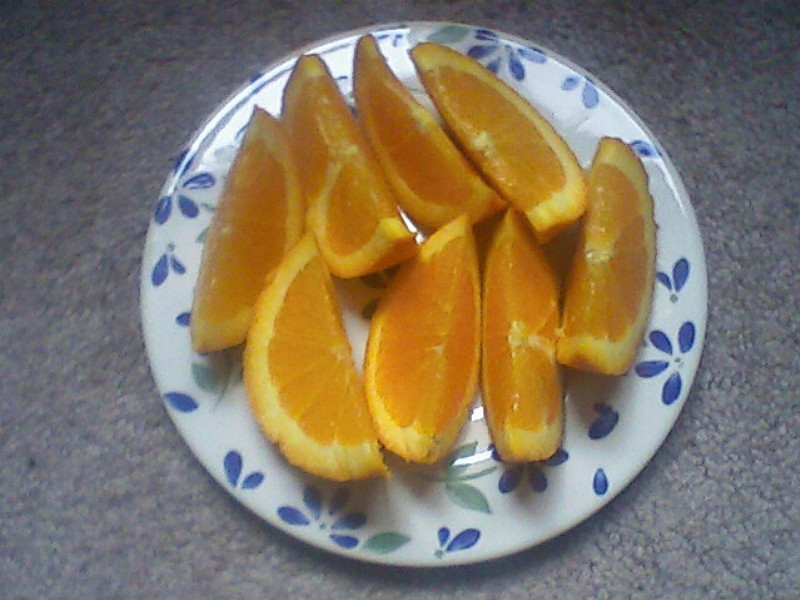A photograph captures a small, detailed arrangement of orange slices on a picturesque plate, set against a gray surface that features subtle blue or purple veins. The plate itself is white with elegant, watercolor-style cornflower blue petals and light green leaves. On the plate are eight medium-sized orange slices, with their peels still attached. The slices are arranged in two rows of four; the top row and bottom row form a half-circle but are placed somewhat haphazardly, with one bottom slice jutting into the upper row. The bright, shiny orange slices glisten under the light, highlighting their deep color and the delicate membranes still visible on their surfaces. The entire image, despite being a bit grainy and blurry, beautifully showcases the vividness and freshness of the oranges against the intricately designed plate.